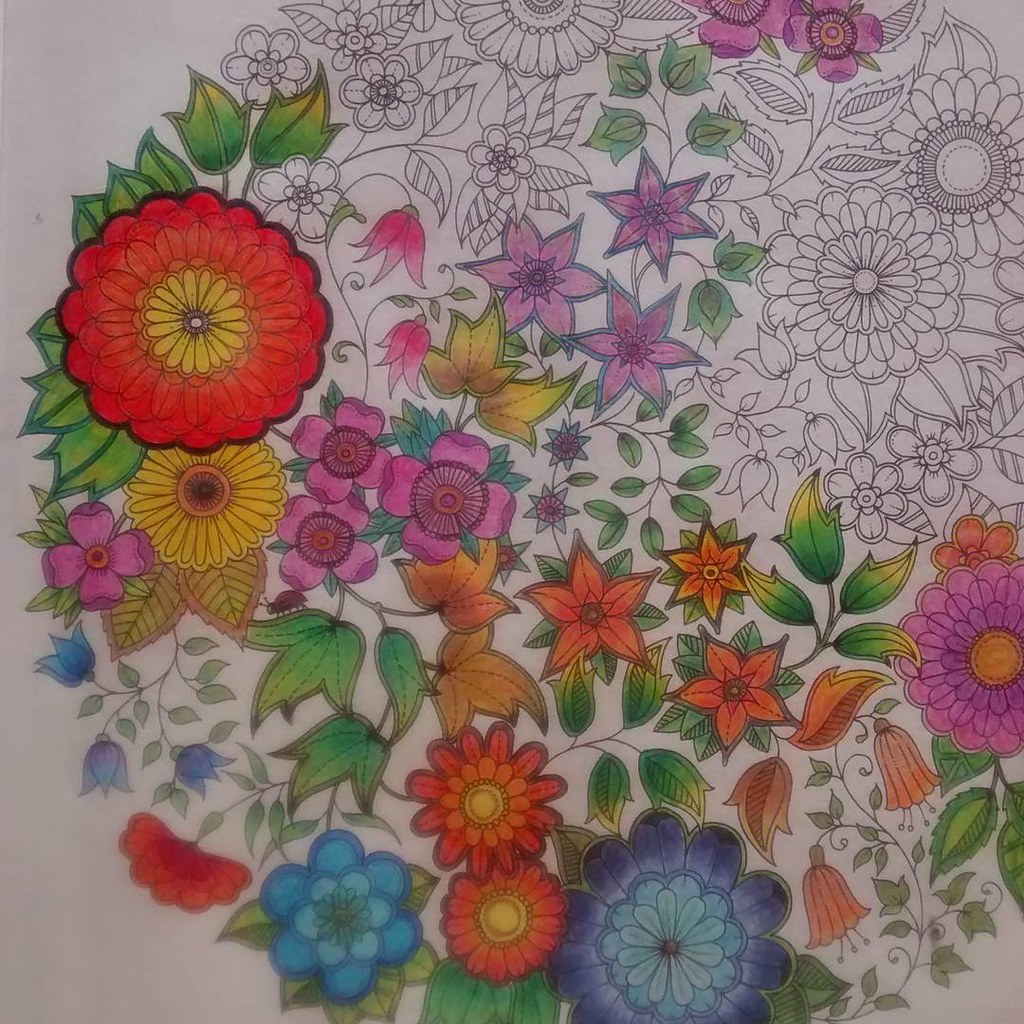The image is a photograph capturing an intricately detailed floral design. The composition showcases a variety of flowers and leaves in a myriad of colors, providing a vivid contrast against a pristine white background. The design appears to be a section of a coloring book, with sections meticulously colored in, while other areas remain in black and white, hinting at printed outlines. 

In the bottom left corner, the abundant use of vibrant shades of green, red, yellow, orange, blue, pink, and purple creates a captivating scene of colored segments. A prominent feature of the design is a large flower situated in the top left corner, boasting bright orange petals and a sunny yellow center. The surrounding flowers vary in hue, adding to the composition's overall richness and diversity. The combination of the hand-colored area with the printed and uncolored segments enhances the artistic allure, presenting a beautifully balanced and visually engaging floral tableau.